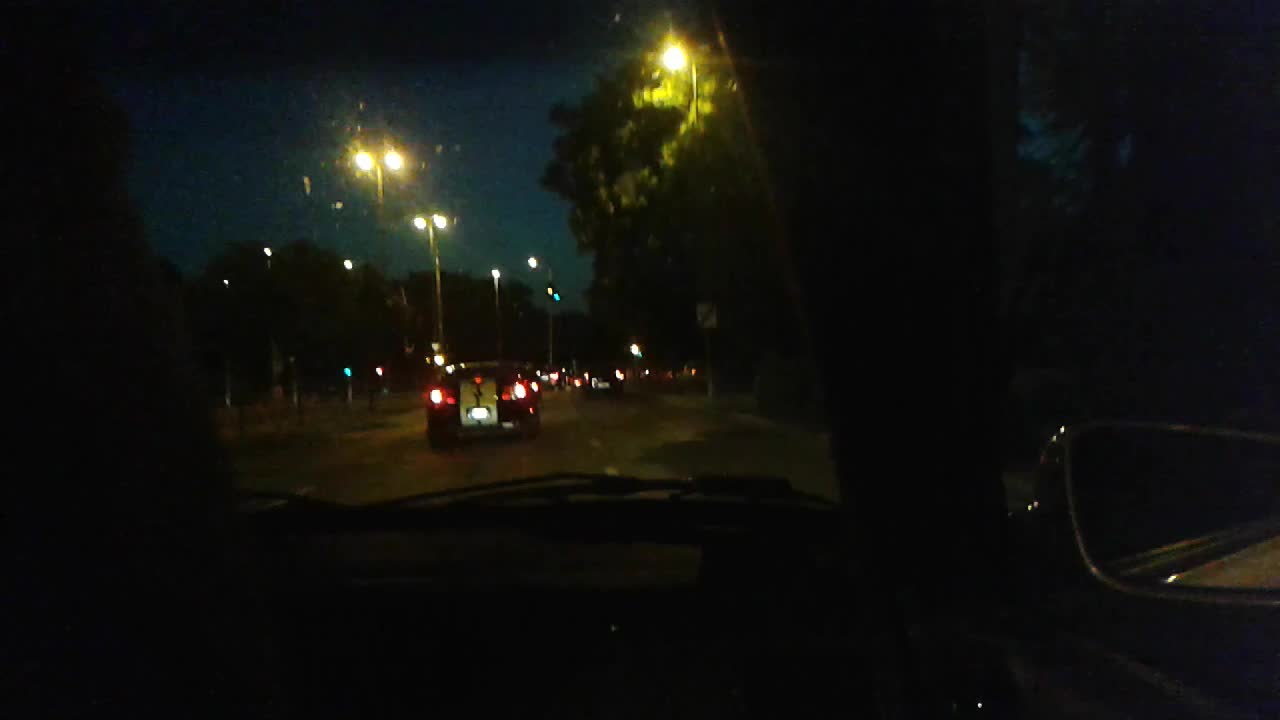This photograph, taken from the passenger side of a vehicle, provides a detailed view through the car's windshield. On the right side of the image, the rearview mirror is visible, along with a portion of the dashboard and the windshield wiper extending across the glass. The dark, slightly visible post separating the window and the windshield adds depth to the composition. 

The scene outside showcases a gray, three-lane road marked with dotted white lines. Dominating the immediate field of vision is a car with distinctive white racing stripes down its back, which strongly resembles a Mustang. The vehicle’s red taillights are glowing, contributing to the nighttime ambiance.

Ahead, a couple of street lamps mounted on silver poles cast a bright yellow light onto the scene. Flanking the road, trees stand illuminated in a vivid green, contrasting sharply against the nearly black background, creating an intriguing interplay of light and shadow.